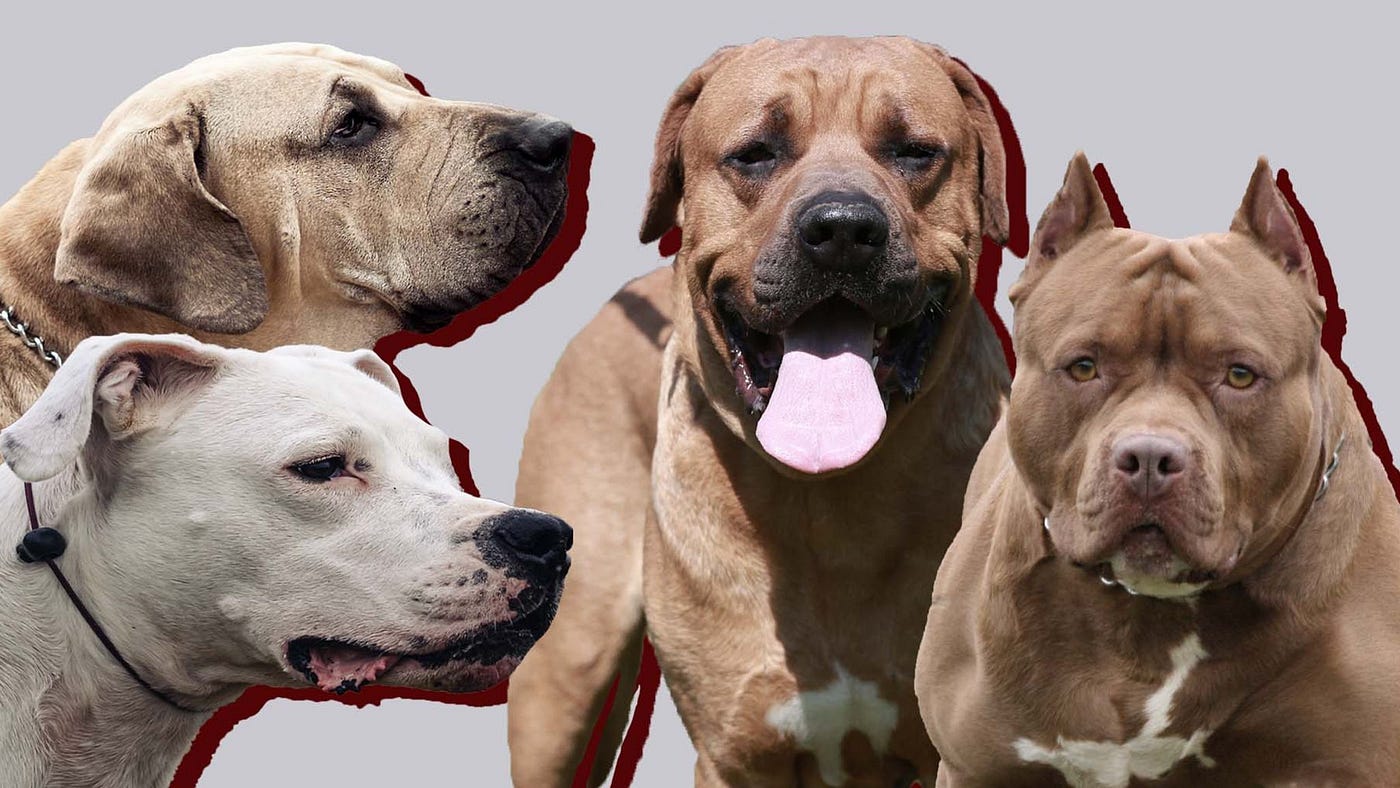In a landscape layout image with a grey background, four different types of pitbulls are showcased in a detailed and cohesive arrangement. On the right side, a muscular light brown pitbull with pointy, docked ears and golden brown eyes stands out, sporting a silver chain around its neck. Next to it, a similarly beige-brown pitbull with a black nose and a pink tongue hanging out strikes a friendly pose. On the left side of the image, there are two pitbulls with only their heads visible, layered one above the other. The upper dog, in profile, features a light yellowish-brown hue with a brown nose and another silver chain collar around its neck. Below, a white pitbull head with black eyes and nose and a black collar also looks out in profile. This composition of differently posed pitbulls highlights their varied sizes, colors, and distinctive features.